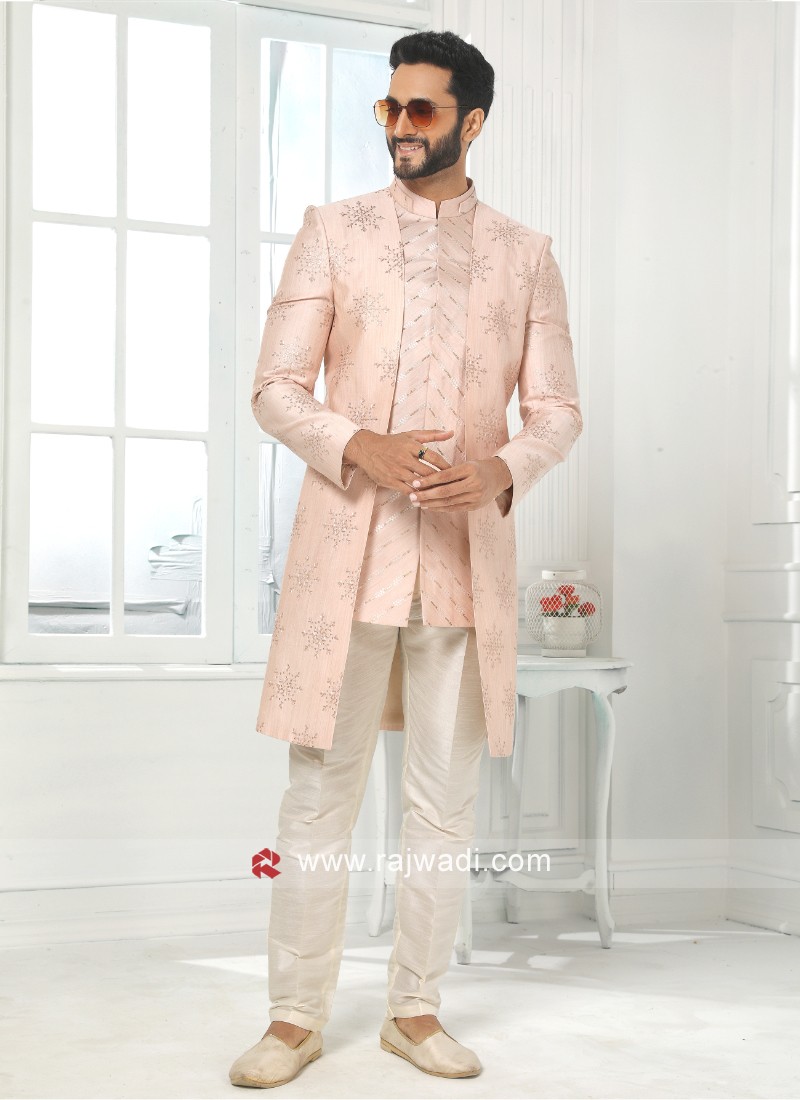In the center of the image, a man stands in a house setting. At the lower portion near his knees, there is a red symbol accompanied by the text "www.rajwadi.com" in white letters. The man is dressed in a pink suit with a matching pink collared undershirt, gray dress pants, and light gray shoes. His hands are positioned at the bottom of his torso, with his right hand gently grasping his left fingers. He is facing slightly to the left, sporting a black beard and hair, a smile, and wearing sunglasses that have a gradient from red at the bottom to black at the top. The room has an entirely gray color palette, including the walls, window frame, floor, and baseboard.